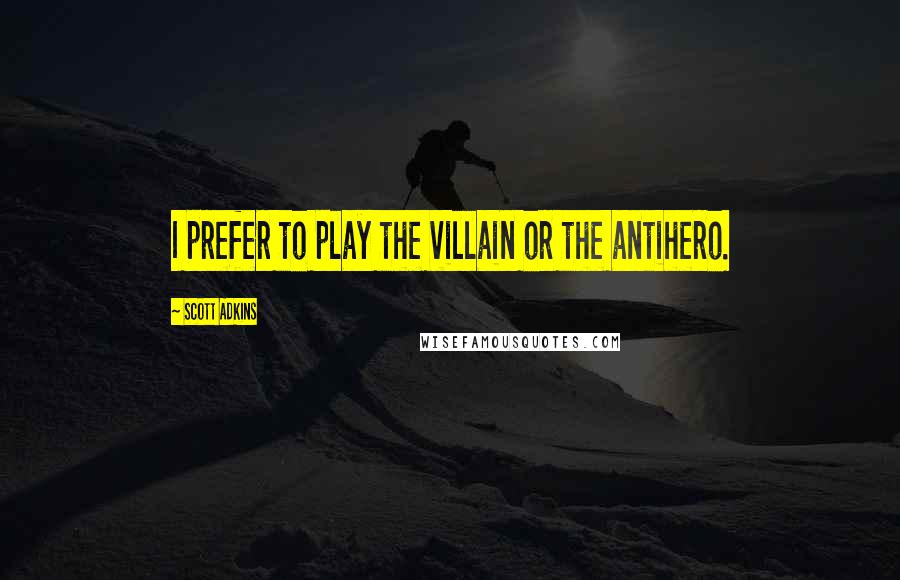The poster features a striking central image of a lone skier descending a snow-covered mountain, with the sun setting in the background, casting a grayish, ominous hue over the scene. The sky is tinged with hints of blue and scattered clouds. A yellow banner with black text prominently stands out in the middle of the poster, displaying the quote: "I prefer to play the villain or the anti-hero." This quote is attributed to Scott Adkins and cited from wisefamousquotes.com. The athlete on skis adds a sense of solitude and adventure to the scene, underpinned by a water body visible toward the right. The bottom section of the poster seamlessly blends into the snowy decline of the mountain, enhancing the overall wintry and remote atmosphere.